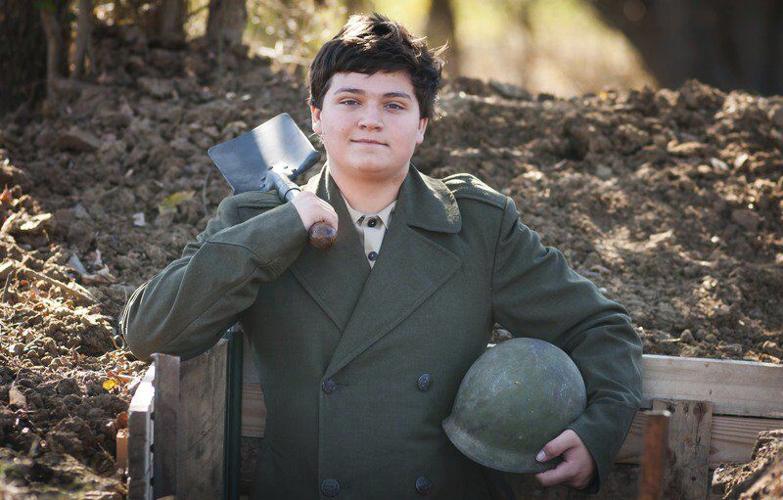The photograph captures a young man with dark hair, standing outdoors in daylight, in front of a wooden retaining wall and a mound of dirt. He gazes directly at the camera with a wry smile on his face. The young man is dressed in a formal military uniform, featuring a dark green double-breasted wool coat and a light khaki buttoned shirt visible beneath it. In his left hand, he holds an olive green helmet with some gray discoloration, while his right hand carries a small hand spade slung over his shoulder. The scene has no text and conveys a sense of historical military representation.